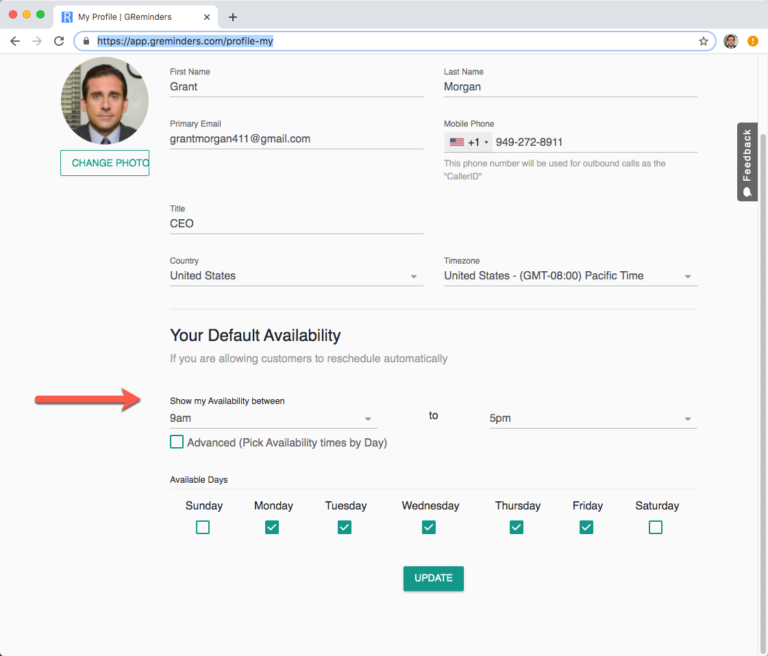This detailed caption describes an image of a Safari browser window on a Mac, displaying the profile page of the GReminders website.

---

The screenshot captures the GReminders profile page accessed through Safari on a Mac, as indicated by the three distinct red, orange, and green buttons in the top-left corner. The web address shown is "https://app.greminders.com/profile-my."

On the profile page, user information is filled out as follows:
- **First Name:** Grant
- **Last Name:** Morgan
- **Primary Email:** grantmorgan411@gmail.com
- **Mobile Phone Number:** Not specified
- **Title:** CEO
- **Country:** United States
- **Time Zone:** United States GMT-08:00 Pacific Time

Below this, there's a section labeled "Default Availability," featuring drop-down menus for selecting AM and PM times. An additional button allows users to access an advanced menu for setting availability times by specific days.

Further down, there's a series of checkboxes for selecting available days of the week. The options are:
- Sunday
- Monday (checked)
- Tuesday (checked)
- Wednesday (checked)
- Thursday (checked)
- Friday (checked)
- Saturday

An "Update" button is present to save any changes made.

A red arrow highlights the text "Show my availability between."

At the top of the page, there's a circular profile picture displaying an image of Michael Scott from "The Office." Directly beneath this image, there's a button labeled "Change your photo" for updating the profile picture.

---

The detailed caption provides a comprehensive and organized description of the screenshot's contents, making the information clear and concise.